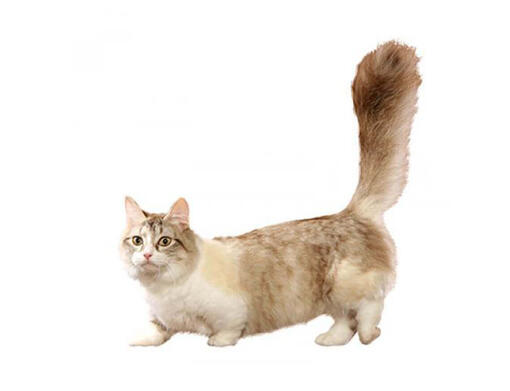This image features an adorable munchkin cat with notably short legs, giving it a distinctive appearance. The cat is crouched slightly to the left, with its fluffy tail held high and prominently in the air. The tail, which is increasingly darker towards the tip, stands out with its dramatic transition from lighter hues near the base to a dark brown at the top. The cat’s cream-colored fur is accentuated with light brown splotches and markings, giving it a striking, calico-like appearance. The chest is pure white, and the face is a mix of light and dark shades, with one side being much lighter and the other having darker markings that echo the tail's coloration. The cat's big, expressive eyes are directed towards the camera, showcasing a hint of eye gunk. It has a very pink nose, and the fur texture looks fluffy yet smooth. The cat is holding its left rear leg slightly up and appears to be in mid-step, enhancing its dynamic and engaging pose. The inside of its ears is tinted pink, adding to its overall charming look.